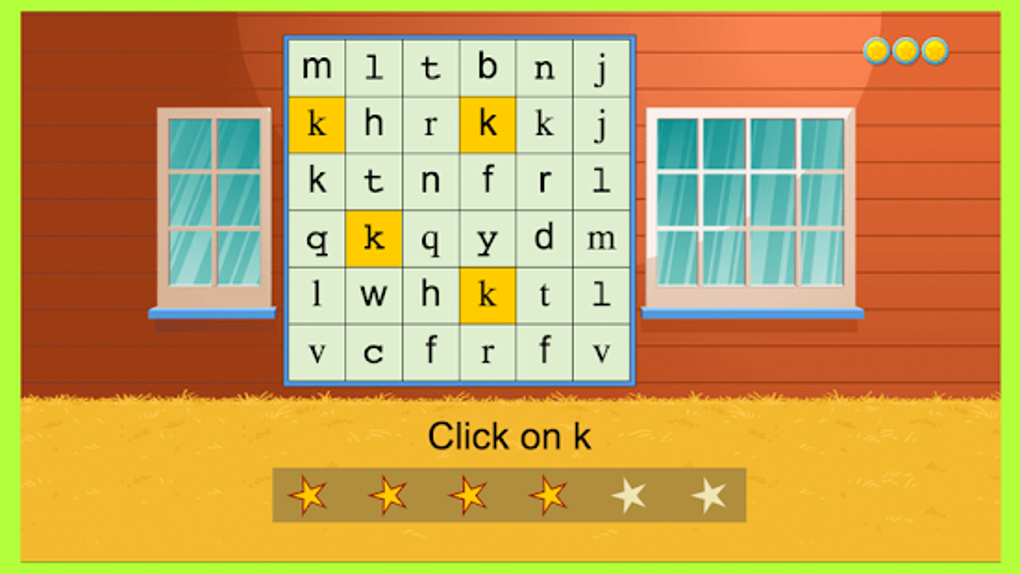This image appears to be a screenshot from an educational game designed to help users identify letters. The game board consists of a grid with six rows and six columns, each cell containing a randomly scattered letter. Among these letters, four instances of the letter 'K' are prominently highlighted in yellow, contrasting against the off-white background of the other cells. Each letter is displayed in black for clear visibility.

The backdrop of this scene resembles the exterior of a rustic barn or house, characterized by brown siding and fitted with two windows, one positioned to the left and the other to the right of the letter board. Below the grid, there is an instruction that reads "Click on K," guiding the user’s interaction with the game. Accompanying this instruction are six stars; the first four stars are illuminated in yellow with a red outline, likely indicating the player's progress or remaining attempts to successfully complete the task.